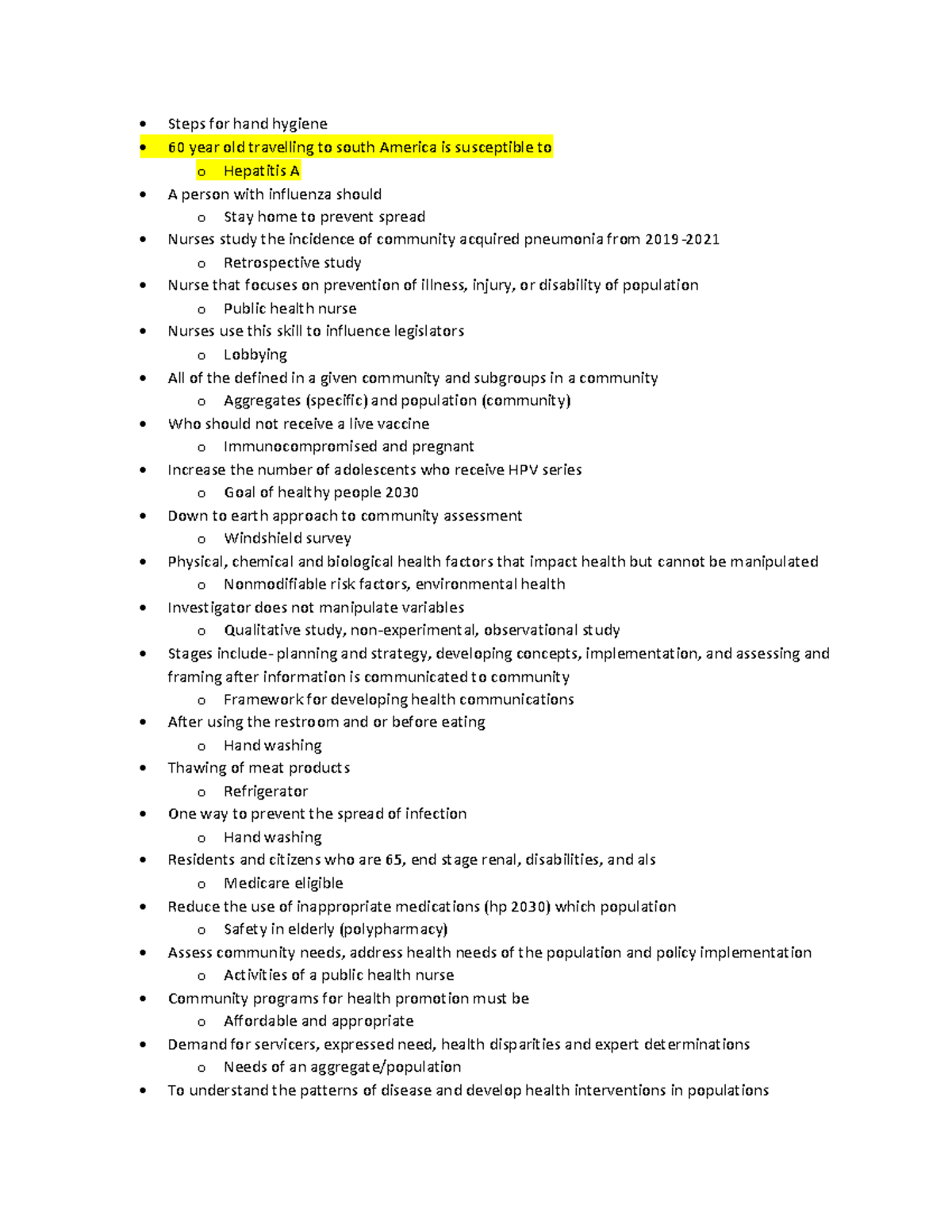The image displays a bulleted communication document, left-aligned, characterized by a series of strategically formatted points. 

1. **Steps for Hand Hygiene**: This entry is marked with a solid black bullet point.
2. **Highlighted Information**: Below, there is a notable section with a yellow highlight stating, *"60-year-old traveling to South America is susceptible to Hepatitis A."* Hepatitis A is referenced again with a circled bullet of white color, distinctively overlaid by the same yellow highlighting.
3. **Influenza Guidance**: Following this, another bullet point states, "*A person with influenza should*," accompanied by clear, unhighlighted text advising individuals to *"stay home to prevent spread."*

In total, the document contains over ten distinct points, with at least three specific references related to nurses, categorized similarly. The background of the document is white, and it lacks both a heading at the top and any definitive conclusion at the bottom.